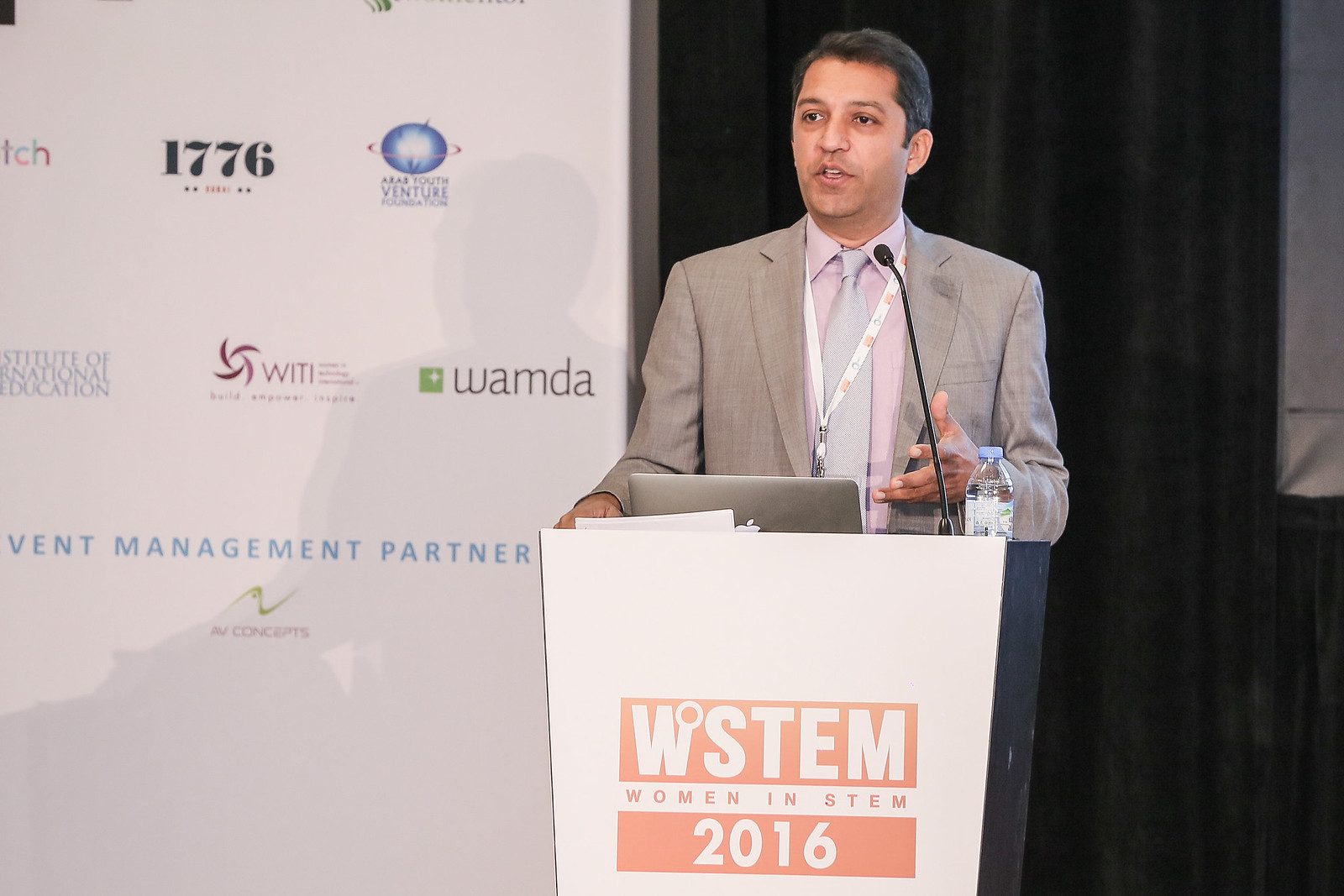In the image, a man stands at a white podium in the center of the frame, speaking into a microphone. The front of the podium displays the text "WSTEM Women in STEM 2016" in distinctive lettering, with "WSTEM" in white on a red background, "Women in STEM" in smaller red letters on white, and "2016" in white on a red horizontal strip. The man, who appears to be of Indian descent, is dressed in a gray suit, a light blue or lavender tie, and a white lanyard around his neck. His left hand is extended in a gesturing manner, while his right hand rests on the podium. A MacBook and a small water bottle are positioned on the upper right corner of the podium. Behind him, a dark gray curtain serves as the backdrop, and to his right, a section of a white barrier features multiple sponsor logos, including "1776," "WAMDA," a blue globe, "Arabs Youth Venture," "WITI," and "VENT Management Partner." The setting, likely indoors, appears to be during a formal presentation or conference.